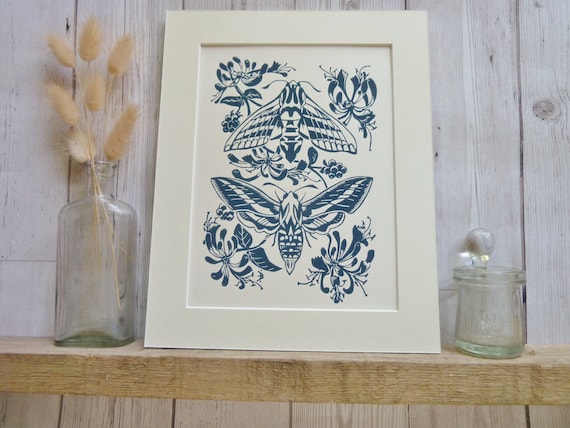The image depicts a meticulously framed painting of two distinctively colored butterflies stacked one above the other, each with their wings spread in opposite directions. The butterflies feature intricate details: the lower butterfly exhibits a blue hue with white accents, while the upper one has a more muted, whitish coloration with dark blue spots. Surrounding the butterflies, the corners of the painting are adorned with dark blue silhouetted florals and berry-laden plants, adding a delicate touch to the composition.

This artwork is set against a white background and is framed by a white mat, further enhancing its elegance. The framed image is positioned on a beige wooden beam that is attached to a whitewashed wooden wall composed of multiple panels, giving a rustic charm to the setting. To the left of the beam, there is an old glass bottle containing strands resembling miniature pampas grass or wheat, adding a natural element. On the right side, a small, empty glass jar with a lid completes the arrangement, creating a harmonious still-life scene.